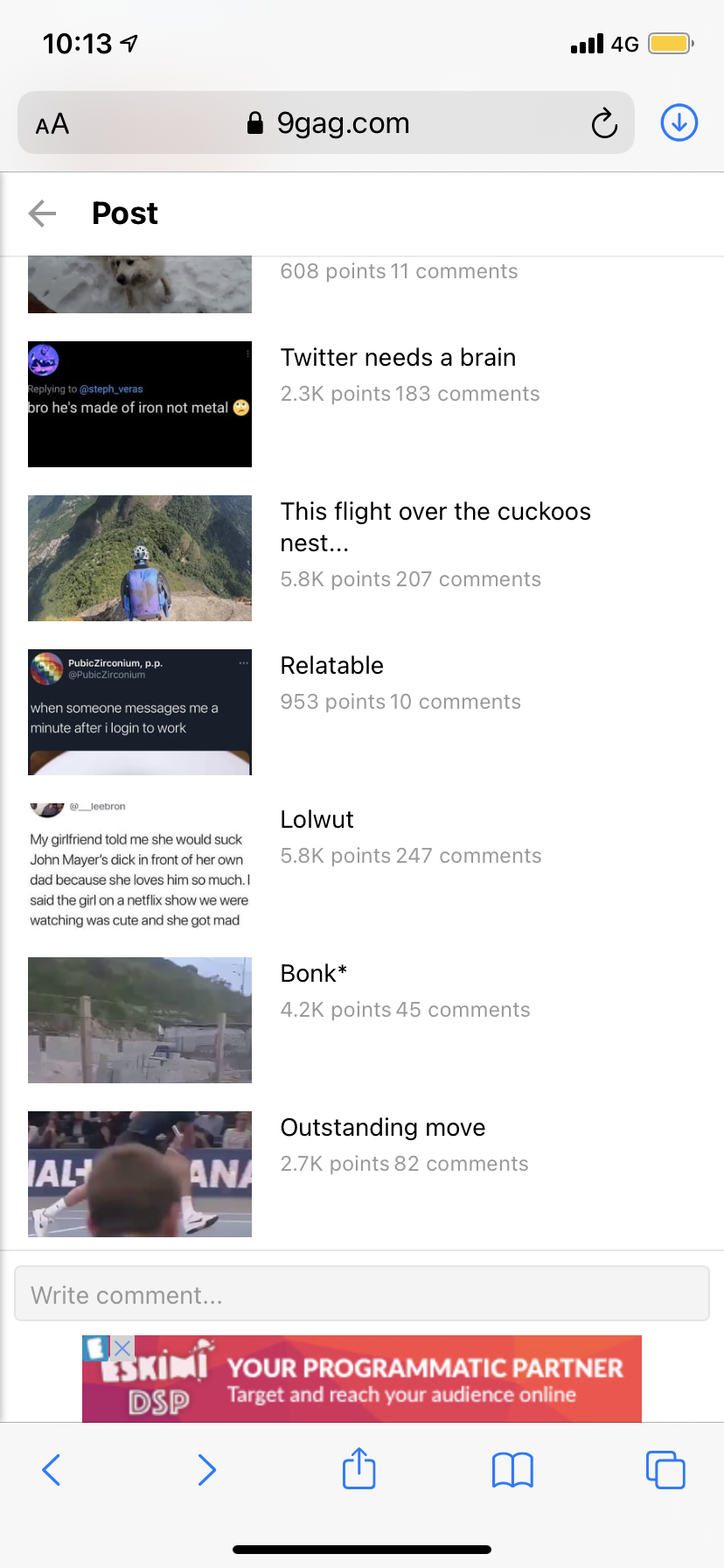This image captures a screenshot from the website 9GAG.com, viewed on an iPhone. The status bar at the top indicates it is 10:13 AM, with a filled yellow battery icon signaling low power mode. The phone has full 4G service, as suggested by the four bars and a visible location symbol.

Displayed on the website are various user posts with their respective engagement metrics. The prominent post at the top reads, "Twitter needs a brain," and has achieved 2.3 thousand points and 183 comments. Following it, the post titled "This flight over the cuckoo's nest" boasts 5.8k points and 207 comments. Another post, labeled "Relatable," has garnered 953 points and has 10 comments. Below it, the post "LOLWUT" is similarly popular with 5.8k points and 247 comments. Next is the post "Bonk" with 4.2k points and 45 comments. The final visible post is "Outstanding move," collecting 2.7k points and 82 comments. At the bottom of the image, there is an advertisement targeting digital marketers, promoting the services of a programmatic partner to reach online audiences.